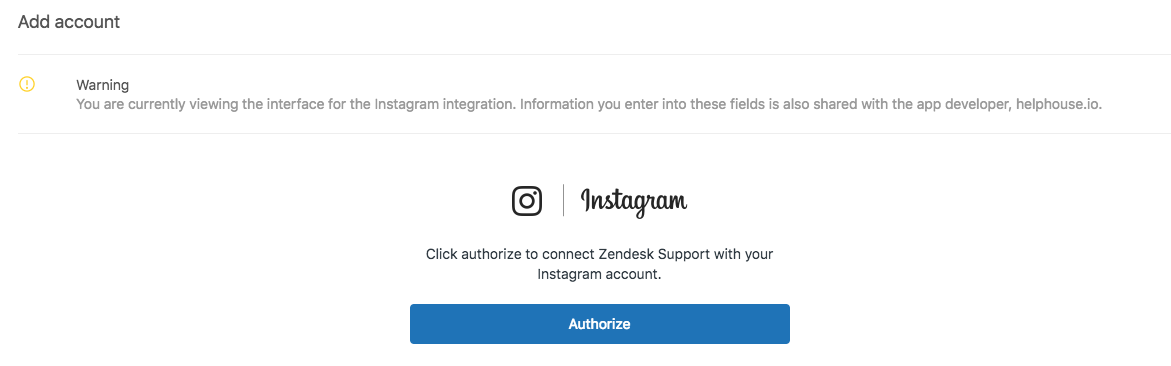The screenshot showcases a minimalist web page with a white background. Positioned at the top left corner, the page features the text "Add Account" in black lettering. Directly beneath this text is a broad, screen-width rectangle in an off-white shade, bordered by a faint gray outline.

In the top left corner of this horizontal bar, there's a yellow circle. Adjacent to the circle, bold black letters spell out a warning: "WARNING: You are currently viewing the interface for the Instagram integration. Information you enter into these fields is also shared with the app developer, HelpHouse.io." 

Below this warning, on the left-hand side, lies the recognizable Instagram icon. To its right, the word "Instagram" is displayed in the familiar cursive Instagram font, written in dark black.

Following this, normal text instructs users to "Click authorize to connect Zendesk Support with your Instagram account." At the bottom of the screenshot, a long dark blue rectangle spans the same width, featuring the word "Authorize" in white letters centered within the blue rectangle.